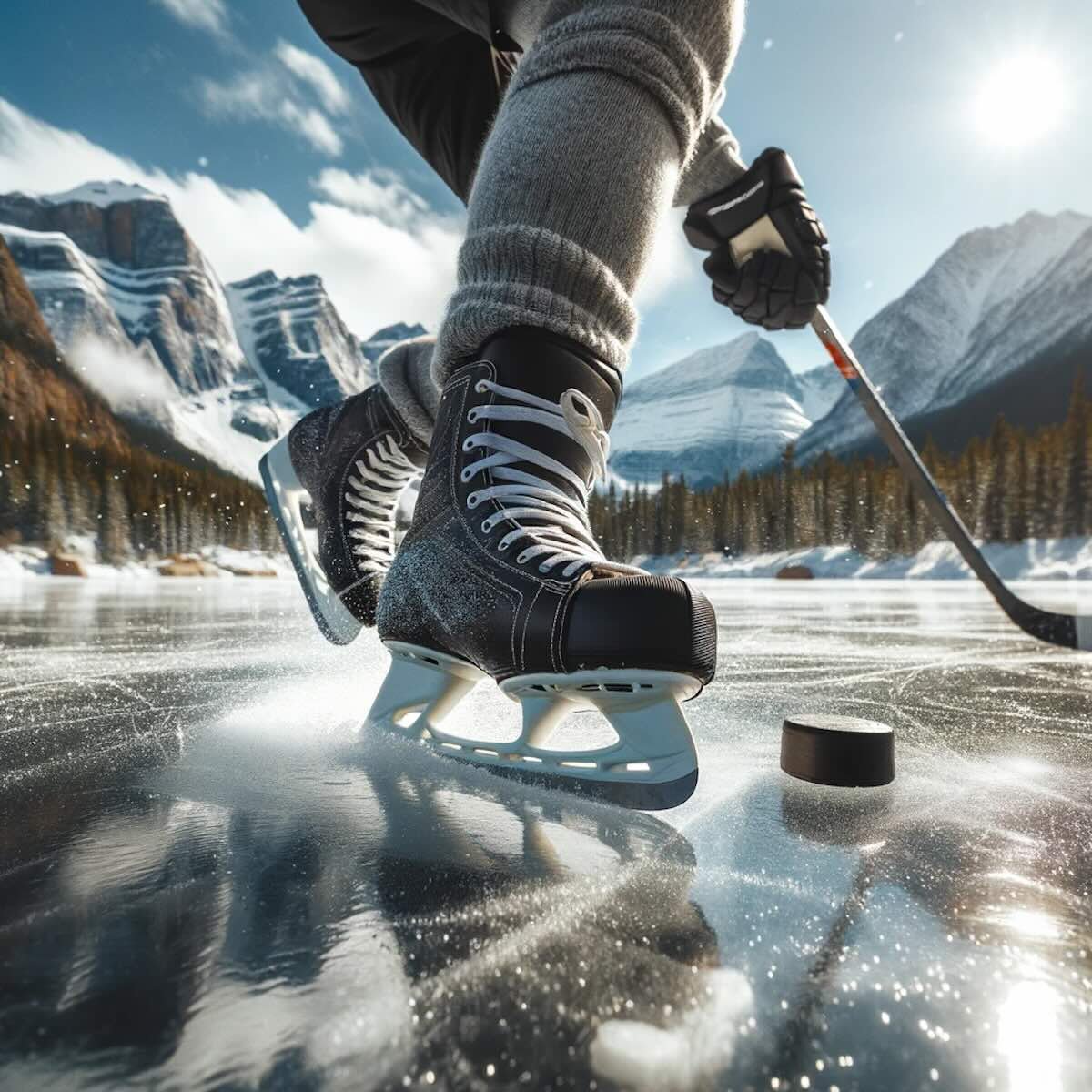The image is a dramatic, close-up photograph of someone playing ice hockey on a frozen pond, captured from a ground-level perspective. The focus is on the skater's legs from the knees down, occupying the central portion of the frame. The skater is wearing black lace-up boots with white laces and long, heavy woolen stockings. The ice is dark and reflective, with visible ice powder dispersing around the skater’s right foot, which is positioned near a black hockey puck as the skater appears to be making a sharp turn. In the skater's gloved hand is a hockey stick. Surrounding the pond is a line of bare trees, and beyond them, jagged mountain peaks rise against a blue sky dotted with clouds and a pale white sun. The overall composition captures the dynamic movement and setting of an outdoor ice hockey game.